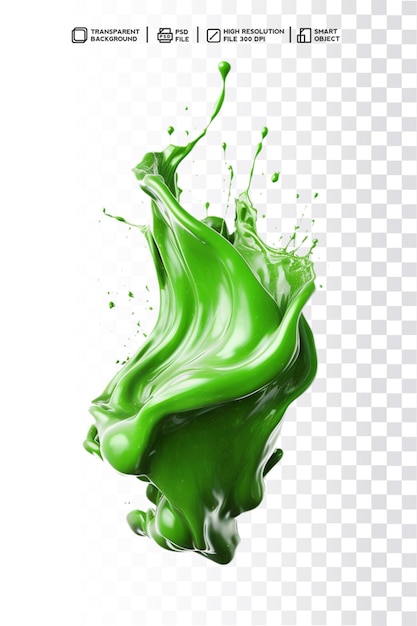This image features a highly detailed and vibrant green liquid, seemingly paint or ink, mid-splash with fluid movements captured in high resolution at 300 dpi. The background showcases a grey and white checker pattern indicating the image's transparency. Text at the top of the image reads "transparent background, PSD file, high-resolution file, 300 dpi, smart object" in black. The green liquid displays a gradient from darker shades at the bottom to lighter hues at the top, likely due to the interplay of shadows and light. The splash forms dynamic ripples as if it is falling apart or spreading out, with additional bits of green debris visible around it.